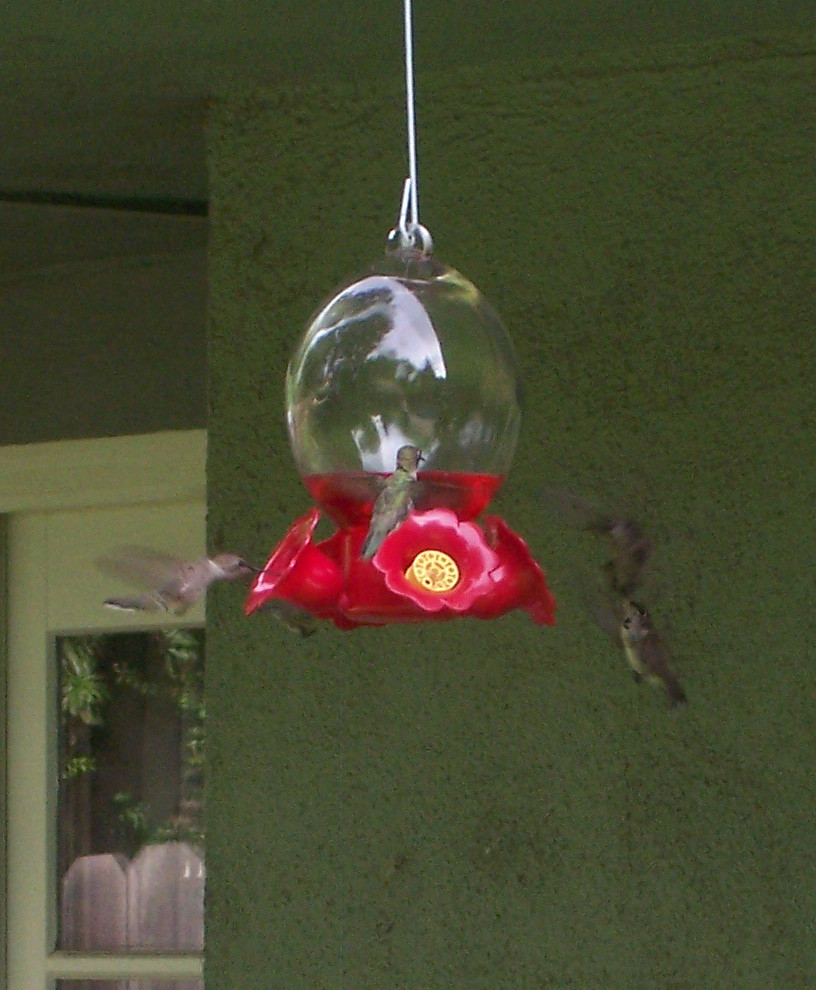The photograph captures a vibrant outdoor scene on a residential porch, featuring a hummingbird feeder hanging from a strong, taut steel wire. The background reveals a painted green stucco wall with a white window, offering a glimpse of reflected leaves from nearby trees and a privacy fence, indicating a bright, sunny day. The hummingbird feeder itself is striking with its red base, clear glass bulb, and artificial red plastic flowers complete with yellow centers, designed to dispense nectar for the birds.

In the foreground, we see the detailed yellow plastic holders with slots for the hummingbirds' beaks. One of these artificial flowers faces the camera, capturing a hummingbird mid-hover with its thin beak poking into a flower's slot. Another hummingbird is perched on the flower, adding a touch of stillness amidst the flurry of activity. While the image attempts to capture all the hummingbirds, their rapid wing movements result in a blurred, almost translucent effect with multiple edges, emphasizing their speed and agility. The birds, primarily muted brown with a hint of green, blend into the vibrant scene, with a total of four hummingbirds either flying around or engaging with the feeder. Despite the image's graininess, the dynamic interplay of natural and artificial elements delivers a rich and lively visual narrative.